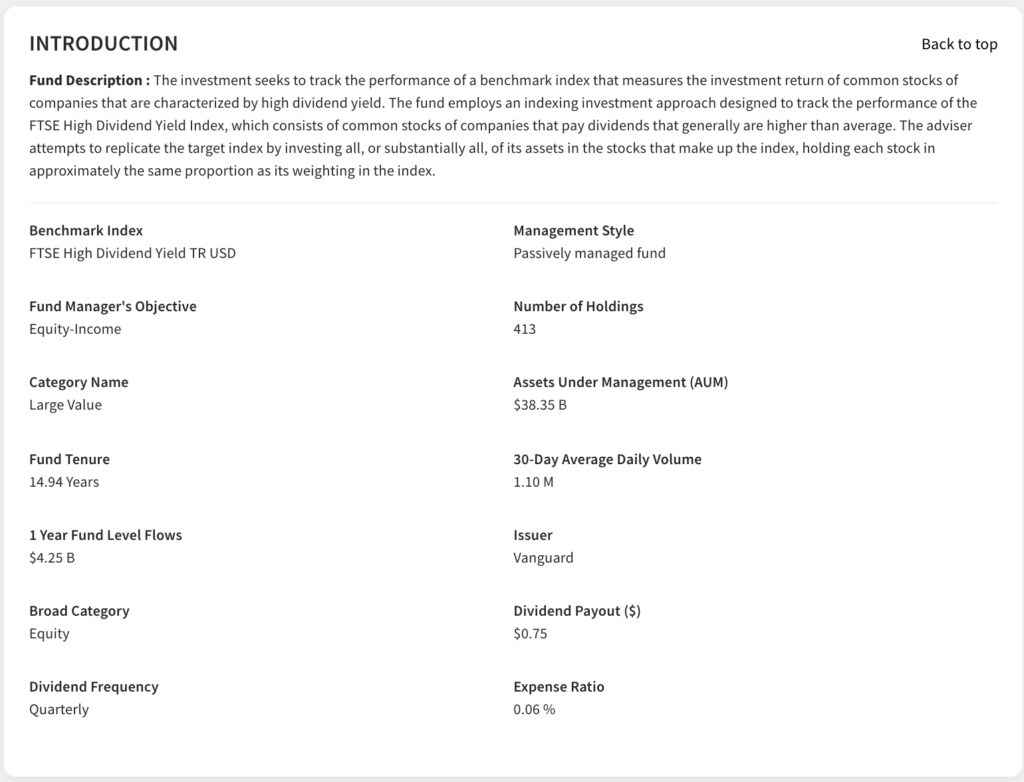Image Caption:

The image displays an investment fund introduction page for the Vanguard High Dividend Yield Index Fund. The fund is designed to track the FTSE High Dividend Yield Index, which includes common stocks of companies known for paying higher-than-average dividends. The fund adopts a passive management approach, attempting to replicate the target index by investing most of its assets in the same stocks and in similar proportions as the index. With an equity income objective and categorized under Large Value, the fund has a tenure of 14.94 years and has seen a one-year fund level flow of $4.25 billion. Broadly categorized under Equity, it pays dividends quarterly and boasts a low expense ratio of 0.06%.

As of the information provided, the fund manages assets worth $38.385 billion and holds 413 different stocks. The 30-day average trading volume is 1.110 million shares, with a current dividend payout of $0.75 per share, quarterly. The fund is backed by the financial services company, Vanguard. The page layout includes a "Back to Top" button on the upper right-hand side, ensuring easy navigation for the reader.